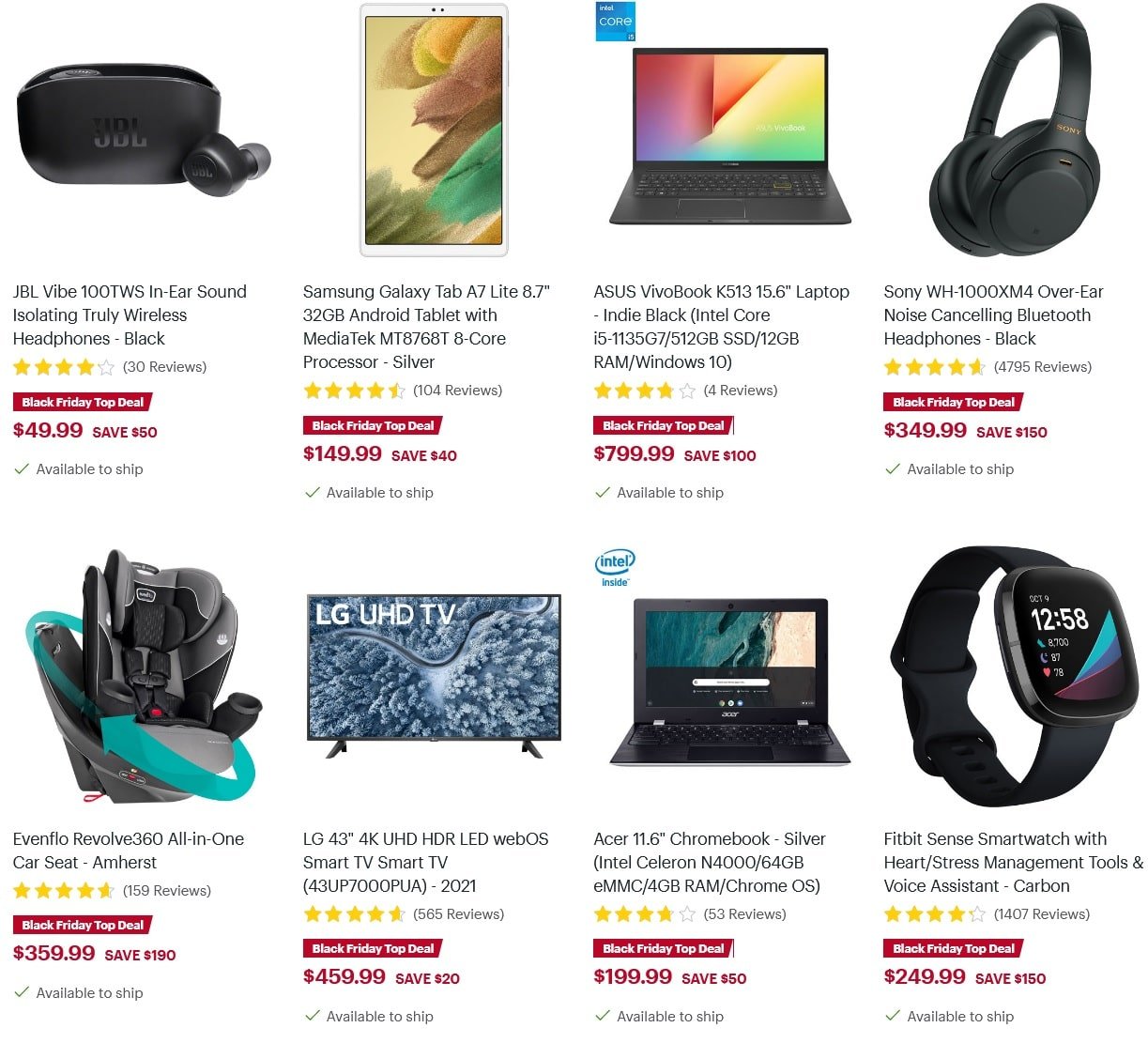This image showcases several advertisements for electronic products, each featuring detailed pricing and customer review information. Here’s a detailed description of each item presented in the image, with highlighted features and current discounts:

1. **LBL Vibe 100 TWS In-Ear Sound:**
   - Visual: Black device with a grey tip.
   - Reviews: ★★★★☆ (30 reviews)
   - Price: $49.99 (red box indicating a $50 saving)

2. **Samsung Galaxy Tab A7 Lite 6.7-Inch:**
   - Visual: Tablet or phone.
   - Reviews: ★★★★☆ (104 reviews)
   - Price: $149.99 (red box indicating a $40 saving)

3. **Laptop:**
   - Visual: Standard laptop.
   - Reviews: ★★★★☆ (4 reviews)
   - Price: $799.99 (red box indicating a $100 saving)

4. **Earphones:**
   - Visual: Standard earphones.
   - Reviews: ★★★★☆ (47 reviews)
   - Price: $349.99 (red box indicating a $150 saving)

5. **Car Seat:**
   - Visual: Blue arrow making a circle around it.
   - Reviews: ★★★★☆ (159 reviews)
   - Price: $359.99 (red box indicating a $190 saving)

6. **LG UHD TV:**
   - Visual: TV displaying "LG UHD TV".
   - Reviews: ★★★★☆ (585 reviews)
   - Price: $459.99 (red box indicating a $20 saving)

7. **Laptop:**
   - Visual: Standard laptop.
   - Reviews: ★★★★☆ (53 reviews)
   - Price: $199.99 (red box indicating a $50 saving)

8. **Smart Watch:**
   - Visual: Standard smart watch.
   - Reviews: ★★★★★ (1407 reviews)
   - Price: $249.99 (red box indicating a $150 saving)

Each product is accompanied by its respective review ratings, showcasing customer satisfaction, while the bold red price tags highlight the savings available on each item.